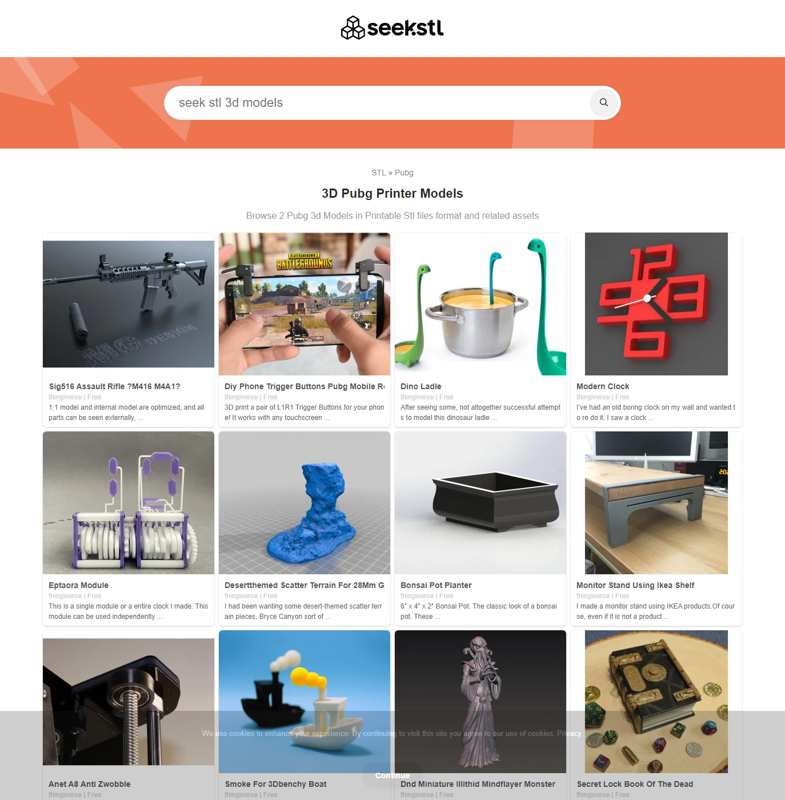The image is a slightly taller than wide square. At the top, the background is white, featuring a logo of three 3D cubes stacked in a triangular formation. To the right of the logo, "seekstl" is written in lowercase letters without spaces. Below this, there is an orange banner with the text "Seek All 3D Models" in the center; this area includes a search box with a magnifying glass icon on the right.

Continuing downwards, the background turns white again. The text "3D PUBG Printer Models" is prominently displayed, followed by a smaller, gray subtitle: "Browse to PUBG 3D Models in printable STL files, format, and related assets." This subtitle is quite small and difficult to read.

Graphically, the main section of the image displays a 4x3 grid of 3D model results. These include an assortment of objects: an assault rifle, a cell phone, a pot, a red clock, what appear to be a couple of baskets, a blue sculpture resembling a melted foot, a black pot, the side of a gray and wood bench, a metal corner piece with a bolt, two ships (one black and one gray), a gray statue, and a book.